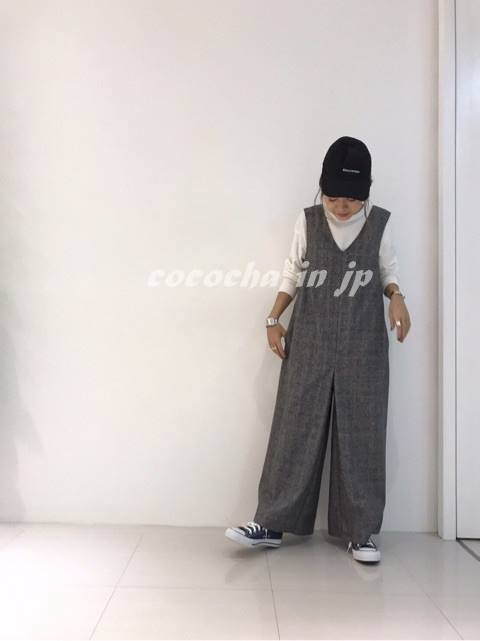In this photograph, a young woman stands against a pristine white wall, showcasing her stylish outfit. Her attire includes a baggy, grayish plaid jumpsuit, which covers her from her feet to above her shoulders, paired with a long-sleeved white dress shirt. On her feet, she sports classic black and white Converse sneakers. She wears a black baseball cap with white text on the front, although the specific words are indiscernible. Her face is tilted downward, slightly smiling, and the sides of her hair peek out from under the cap. Both of her hands display watches and rings, with the left foot slightly raised off the ground. The background features a white gradient wall with large, square white tiles on the floor. On the left, shadows suggest the presence of a house plant outside the frame, while the right side shows a plain white door frame. Etched into the image like a watermark are the letters "C-O-C-O-C-H-A-J-I-N-J-P," possibly denoting the author or photographer.